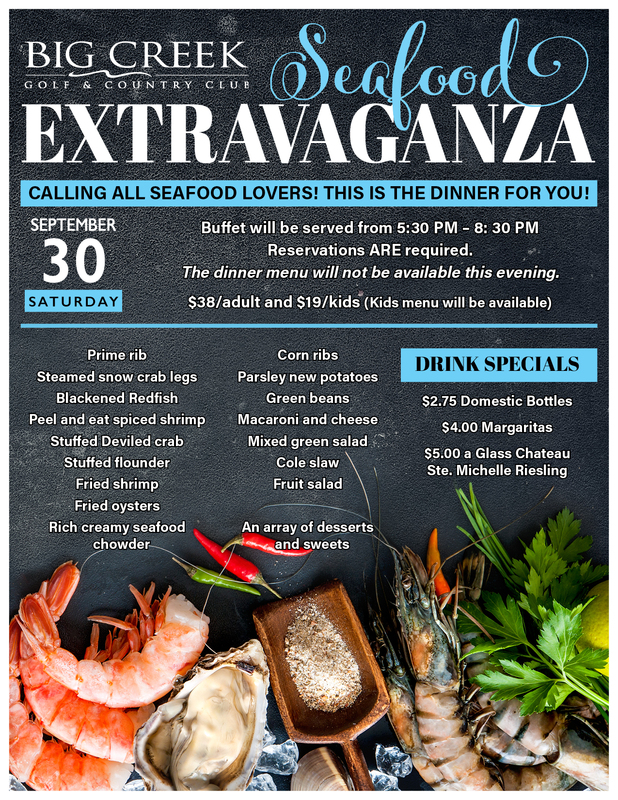The advertisement showcases a visually appealing digital flyer for Big Creek Golf and Country Club's "Seafood Extravaganza." Set against a dark blue or black cutting board-style background, the bottom portion of the image features an enticing array of seafood, including shrimp, open oysters, lobster tails, cilantro sprigs, a wooden scoop of grains, and chili peppers.

In the top left corner, bold white and blue premium text announces the event details: "Big Creek Golf and Country Club Seafood Extravaganza." Beneath this, it reads, "Calling all seafood lovers, this is the dinner for you." The event is scheduled for Saturday, September 30th, with a buffet available from 5:30 p.m. to 8:30 p.m. Reservations are required, as the regular dinner menu will not be available that evening. Pricing is set at $38 per adult and $19 per child (with a kid's menu).

The menu boasts a lavish spread, including prime rib, steamed snow crab legs, blackened redfish, peel-and-eat shrimp, double crab, stuffed flounder, fried shrimp, fried oysters, seafood chowder, corn ribs, and green beans. Drink specials are also listed, featuring $2.75 domestic bottles, $4 margaritas, and $5 glasses of Chateau Ste. Michelle Riesling. This eye-catching promotional poster is ideal for both print and social media, inviting patrons to indulge in a luxurious seafood buffet at the country club.